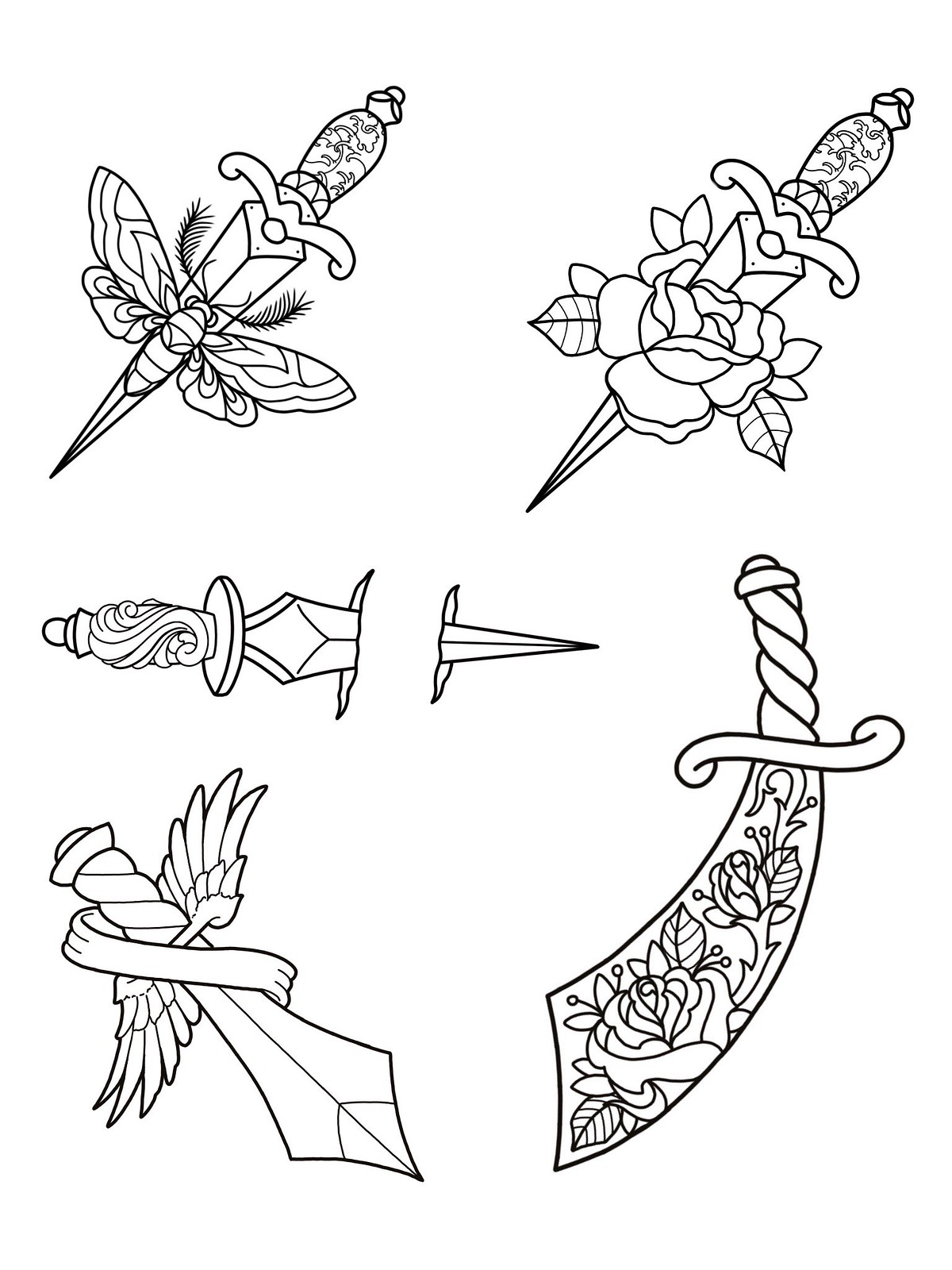This is a black-and-white line drawing, reminiscent of a coloring book or potential tattoo designs, set against a white background with intricate black ink details. There are five dagger-like swords depicted. At the top, two daggers slant diagonally from the left to the upper right, featuring identical ornate handles with what appear to be cloud-like designs; one blade has a butterfly motif, and the other boasts a rose design.

In the center, a horizontally placed sword bisects the image as if cutting through the surface, with a decorative swirling handle. Below this, on the left, a dagger is angled with a winged hilt and a draped banner, adorned with floral elements including roses and leaves. Its handle is twisted and curves elegantly. On the bottom right, just above the center, lies a sword with a spiraled handle, curving blade, and intricate rose embellishments along its length. The detailed and ornate nature of each sword's design makes them potential inspirations for tattoo art.